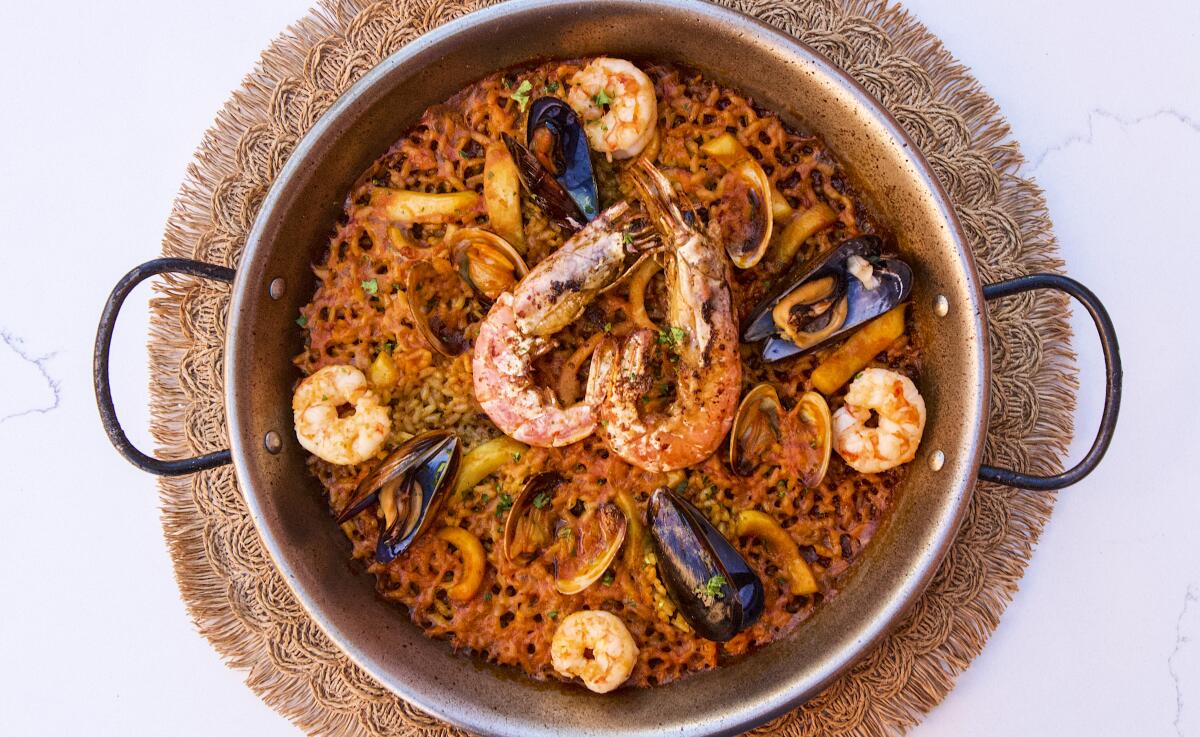An overhead view of a silver paella pan with two black handles, resting on a large circular brown woven doily placemat with fringe, set against a white marble background. The pan contains an orangey-red paella with a variety of seafood. Centered in the dish are large shrimp still in their shells, while along the outer edges, there are shelled shrimp and mussels. The vibrant dish also features a layer of brown and orange rice, with a sprinkle of chopped parsley adding a touch of green on top.